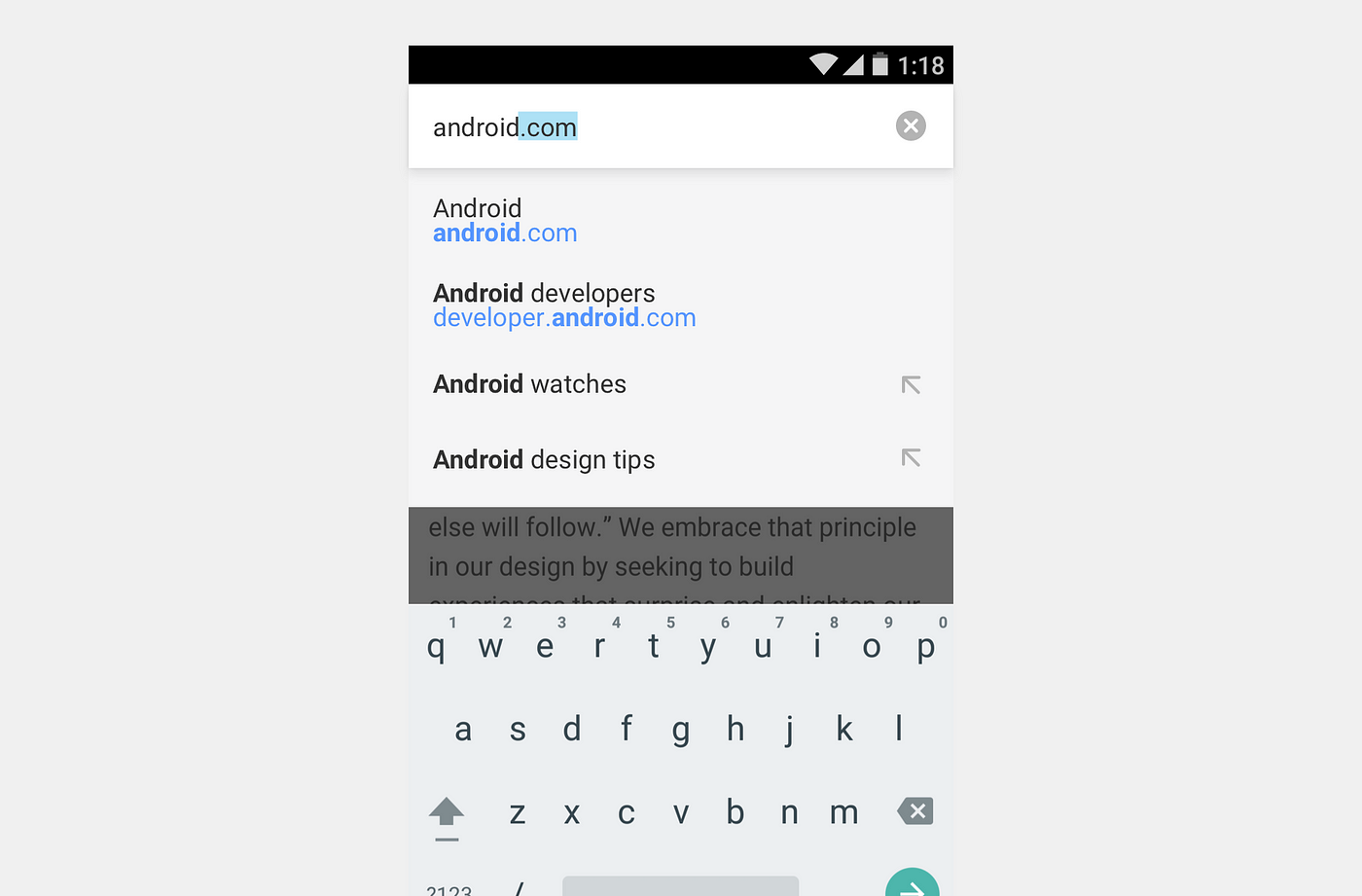This image is a screenshot from a smartphone, presented within a large, very light gray square border. The screenshot’s header area features a background color that is black or possibly a very dark gray. In the top-right corner, it shows the time as 1:18, without specifying a.m. or p.m. Also visible in this corner are the battery icon, the wireless connection icon, and the Wi-Fi icon.

Beneath the header, the background changes to white and forms a white rectangle. On the left side, in gray font, it says "android.com," with the ".com" segment highlighted in light blue. On the right side of this section is a gray circle containing a white "X."

The next section has a background that is a very light gray. Here, the text “android” is in black, followed by "android.com" in blue beneath it. Further down, there are lines of text reading "android developers" in black, and "developer.android.com" in blue. Below these are entries for "android watches" and "android design tips."

A gray rectangle follows, containing black text that reads, "else will follow. We embrace that principle in our design by seeking to build," with the remainder of the text being unreadable. 

The background then transitions to a very light blue where a QWERTY keyboard is displayed in gray letters. The bottom portion of the keyboard is cut off, revealing part of the spacebar and a blue circle with a white right-pointing arrow in the lower right corner, partially out of view.